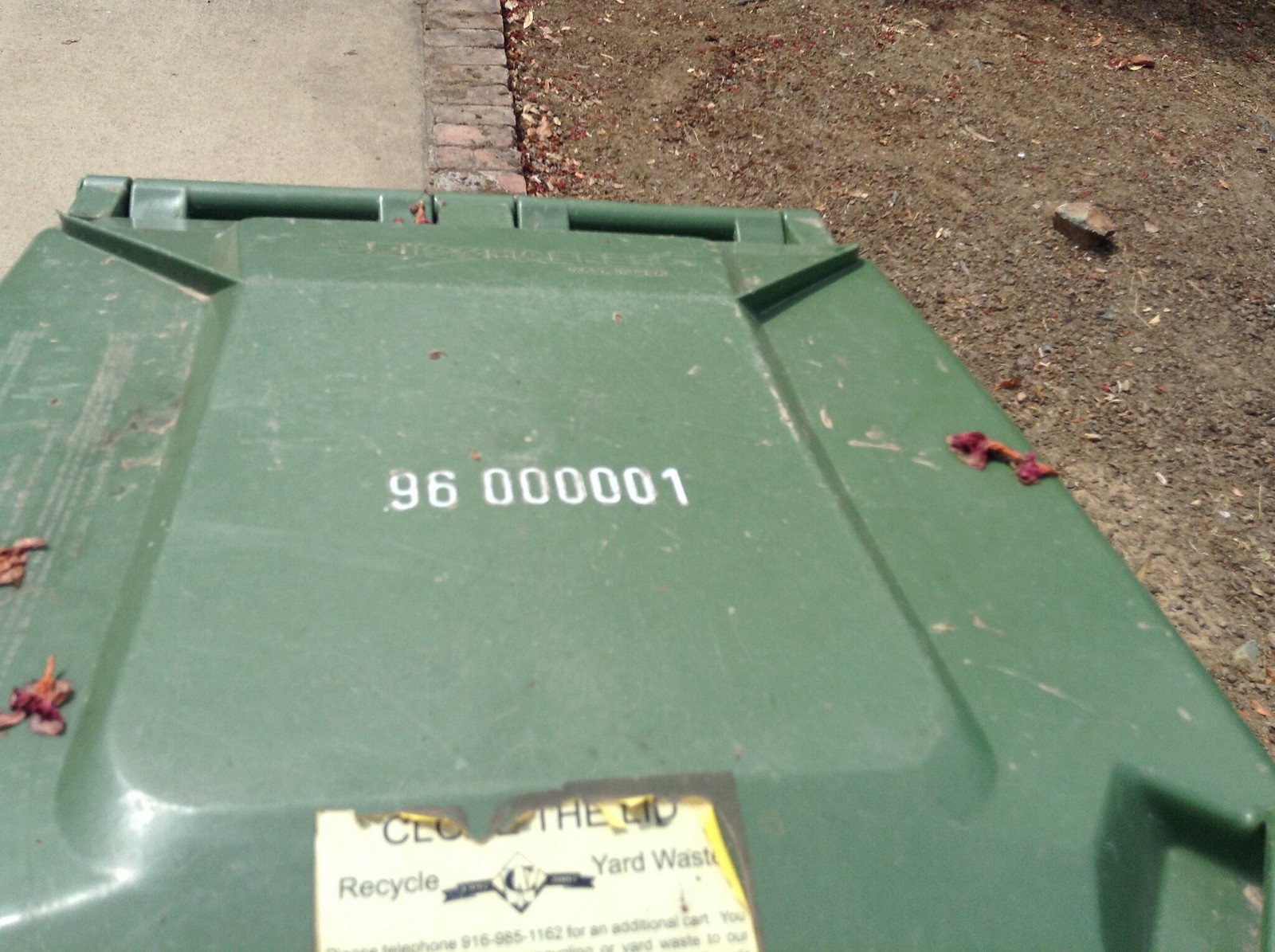Outdoors, the photo captures an army green plastic yard waste bin in the foreground. The top of the bin is littered with dried red flowers and light brown mud smudges. Prominently displayed on the lid are white numerals reading "96000001." A faded and peeling sticker on the edge instructs, "Close the lid, recycle yard waste," though the text is partially obscured. In the background, a dry, brown strip of grass extends across the right half of the image, bordered by a narrow row of bricks. To the left of the bricks lies a gray asphalt walkway. The composition details the interplay between the neglected yard and the functional yet weathered trash bin amidst a blend of natural and constructed elements.